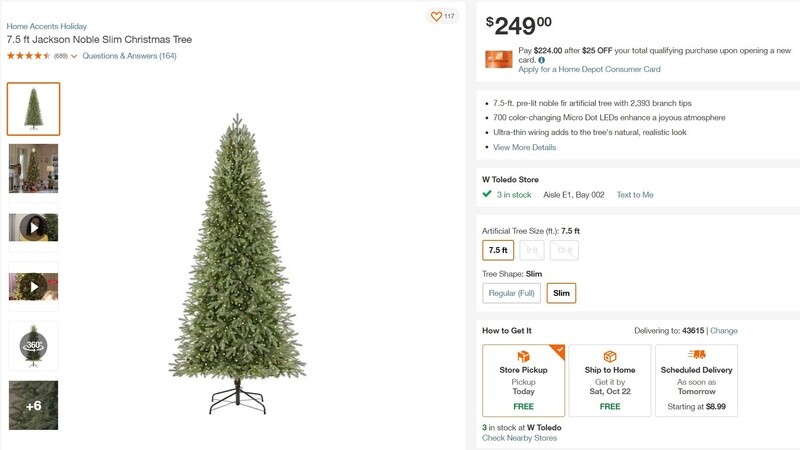The image is a detailed advertisement for a holiday Christmas tree. On the left side, it showcases a 7.5-foot Jackson Noble Slim Christmas Tree available under the Home Accents Holiday brand. The tree has a rating of 4.5 stars from 689 reviews and has 164 questions and answers listed. The main image highlights a close-up of the tree adorned with a yellow box, signifying its selection.

This section also includes various media options such as images and videos. One image shows the tree beautifully set up in a living room, while a 360-degree view feature enables potential buyers to inspect the tree from all angles. Additionally, there are two video thumbnails allowing viewers to watch demonstrations or reviews. An icon indicates there are six or more images available for viewing.

To the right, the advertisement details the price, listing it at $249. It also mentions a special offer: a $25 discount off a total qualifying purchase on opening a new card, which reduces the price to $224. The tree is available in the West Toledo store with three units in stock. It highlights the convenience of multiple delivery options, including shipping directly to the buyer.